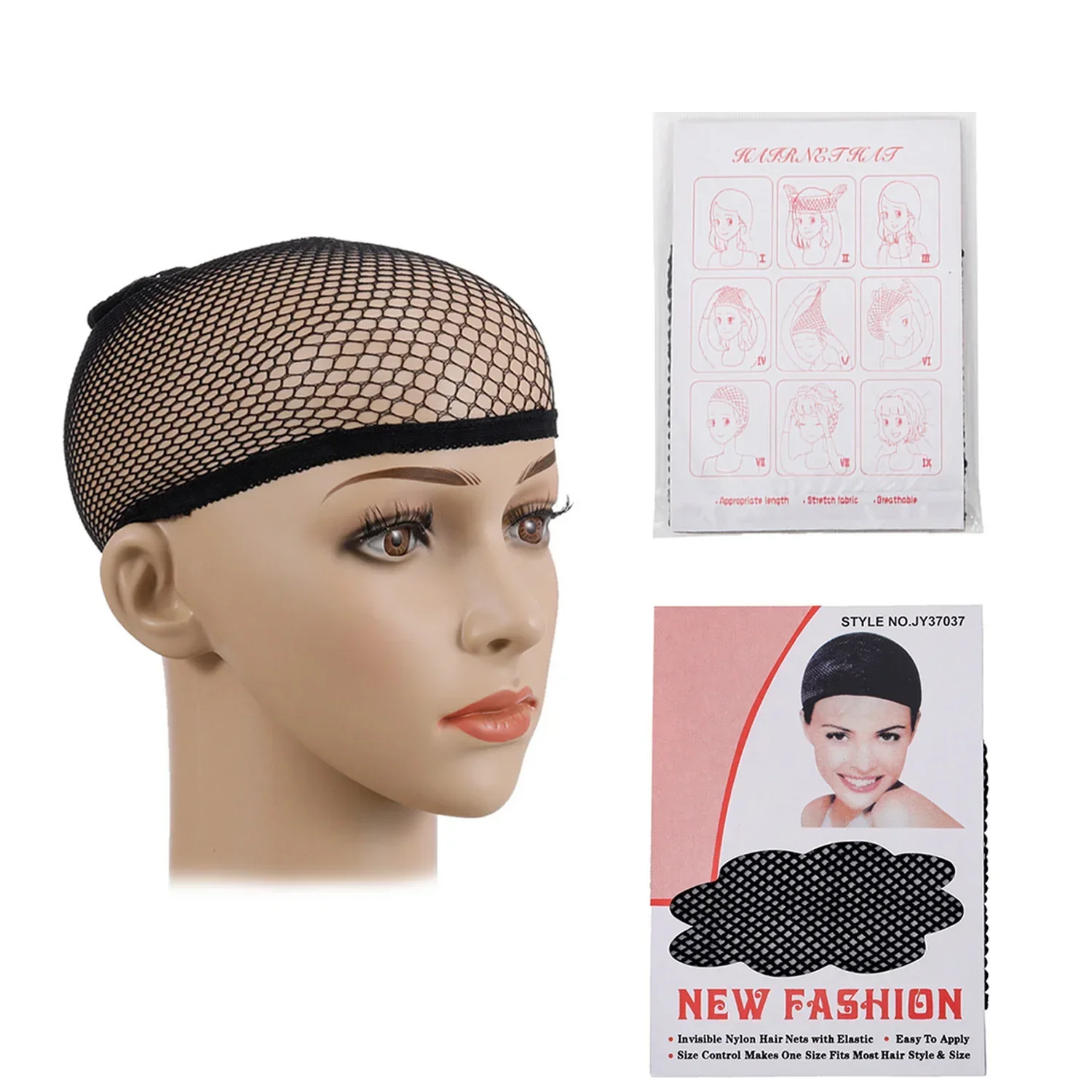The image features the head of a female mannequin on the left side, adorned with a black fishnet hairnet covering its bald head. The mannequin has detailed facial features including eyebrows, long eyelashes, brown eyes, blush on its cheeks, and red lips. On the right side, the top piece of paper displays various hairstyles with a heading that reads "New Fashion," and includes a woman wearing the same fishnet hairnet as shown on the mannequin. Below this, the bottom piece of paper is an advertisement for the hairnet, also titled "New Fashion," showing a model wearing the fishnet and featuring style number JY37037. The advertisement provides instructions for usage, highlighting its versatility for covering natural hair and suggesting it can be easily styled or used as a base for wigs. It mentions that the hairnet is made of stretch fabric, making it a one-size-fits-most product suitable for various hairstyles.